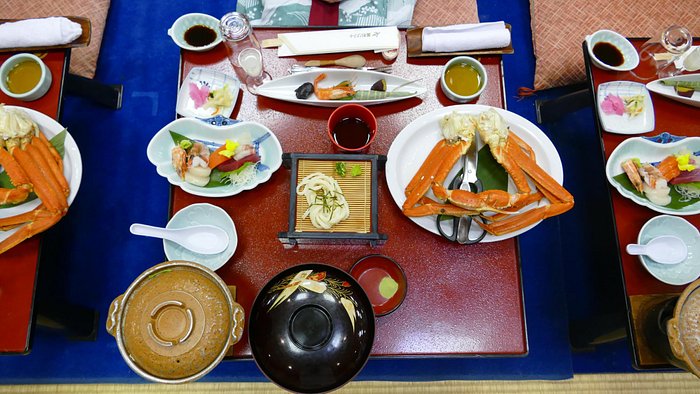This is an aerial photograph of a beautifully arranged Japanese meal, likely taken at a restaurant where guests sit on pillows placed on the floor. The focal point is a large square red tray in the center of the image. On the tray's lower right corner, two covered bowls stand out—one is black with yellow bird illustrations, and the other is a brown pot. To the immediate center-right lies an oblong white plate featuring six neatly arranged crab legs and a pair of kitchen shears with black handles. 

Adjacent to this, more to the center, is a bamboo tray holding a serving of noodles. On the left side of the tray, a selection of sashimi is displayed in elegant Japanese style. There's also some sushi nearby and a couple of pink shrimp positioned at the top of the picture. Completing the setting, chopsticks are placed strategically around the food, which is artistically presented and looks absolutely delicious. The attention to detail and the variety of dishes suggest a meticulously prepared meal meant to impress and satisfy diners.